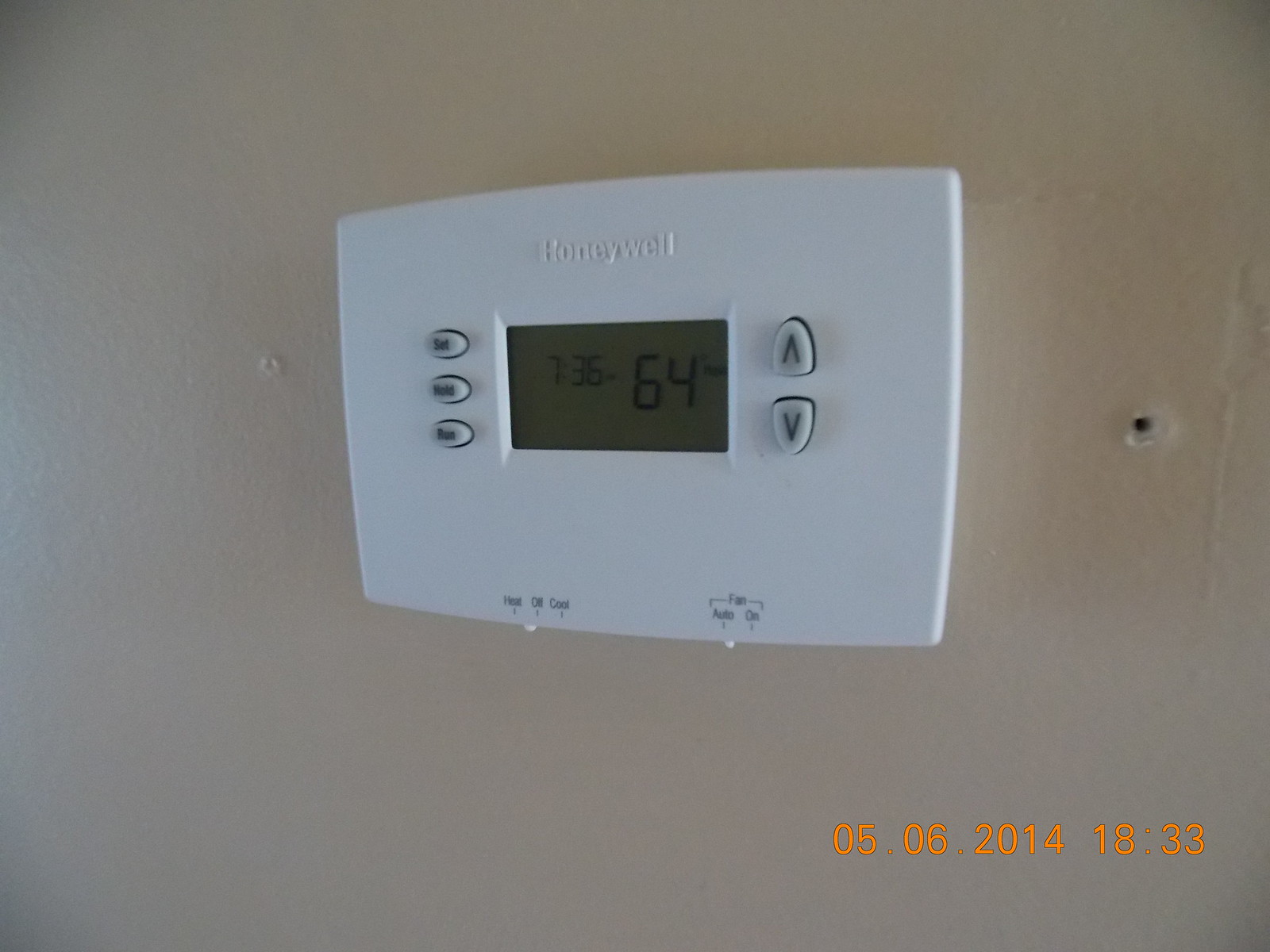In this photograph, the focal point is a close-up of a Honeywell home cooling thermostat. The white, plastic device is mounted on a peach-colored wall and displays a digital clock reading 7:36 PM, although the photograph itself was taken on May 5th, 2014, at 6:33 PM, indicating that the clock might not have been adjusted for daylight saving time.

The thermostat is set to "Auto" mode for the fan, as indicated by the controls at the bottom of the display. The system mode is currently set to "Off," with neither heating nor cooling activated. The current indoor temperature reads 64 degrees Fahrenheit.

Above the temperature display, there are controls labeled "Set," "Hold," and another function that is not clearly visible. These controls allow for the adjustment of the temperature up and down. The device features two visible mounting holes on either side, possibly for screws, contributing to its secure attachment to the wall. The background wall appears as a smooth plaster finish in a peach hue.

Overall, the photograph gives a detailed view of the Honeywell thermostat’s settings and surroundings, highlighting its functional and aesthetic aspects in a home environment.